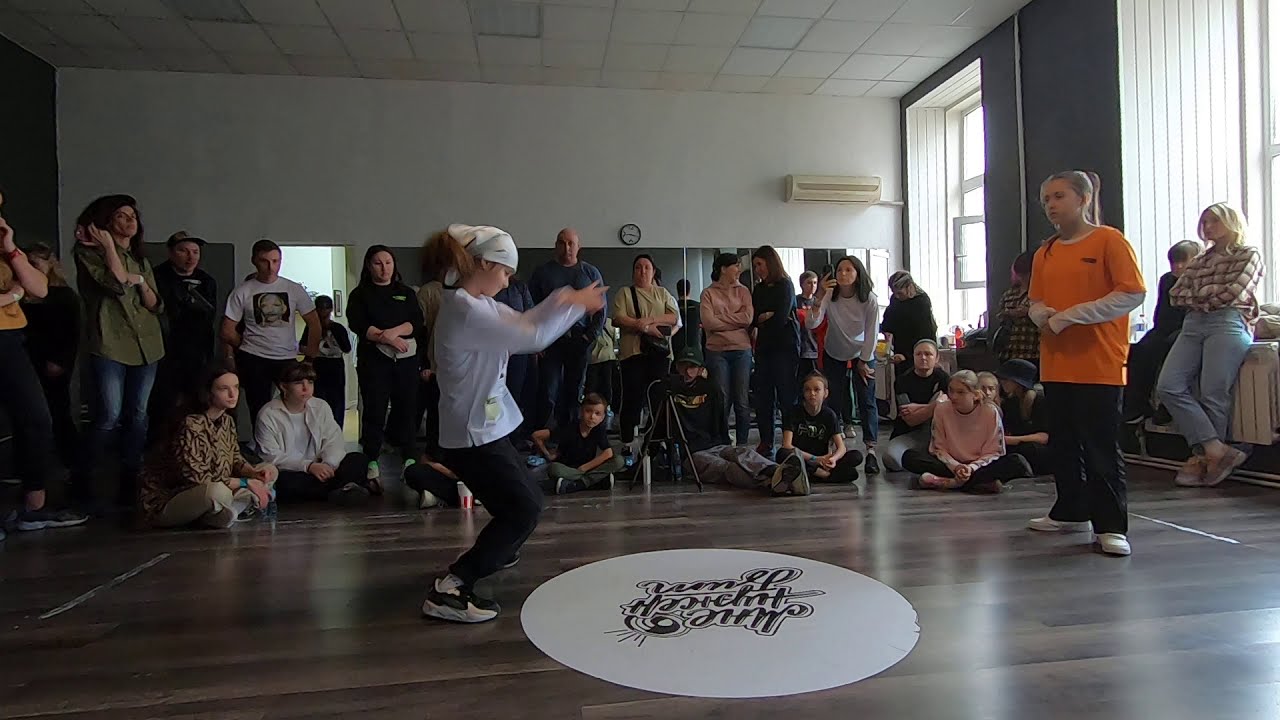In this detailed photograph, you see a group of approximately 30 people gathered in a spacious room that could be an auditorium or gymnasium, characterized by its shiny wooden floor. The focal point of the image is two girls in the middle of the room. The girl at the center appears to be dancing, her legs are bent at the knee, and her arms are raised in the air. She is wearing black pants, white tennis shoes, a white long-sleeve t-shirt, and a white scarf. Her gaze is directed towards the floor. Nearby, another girl stands observing her; she is dressed in an orange top and black pants. At their feet, there is a distinct white circle painted on the floor with black cursive text inside, although the text is difficult to decipher.

Surrounding the two girls, the room is filled with spectators – men, women, and a few children. Some are seated, possibly on the floor or on a radiator by the windows on the right side, while others are standing, forming a line and watching the dance intently. Their serious expressions suggest that the performance holds significant importance. In the background, a long mirror spans the length of the room from one end to the other, extending from a window to an open doorway. Additionally, the back wall of the room is white, punctuated by windows and a clock. The scene is one of concentrated observation, with all eyes trained on the central figure, emphasizing the importance of her movements.